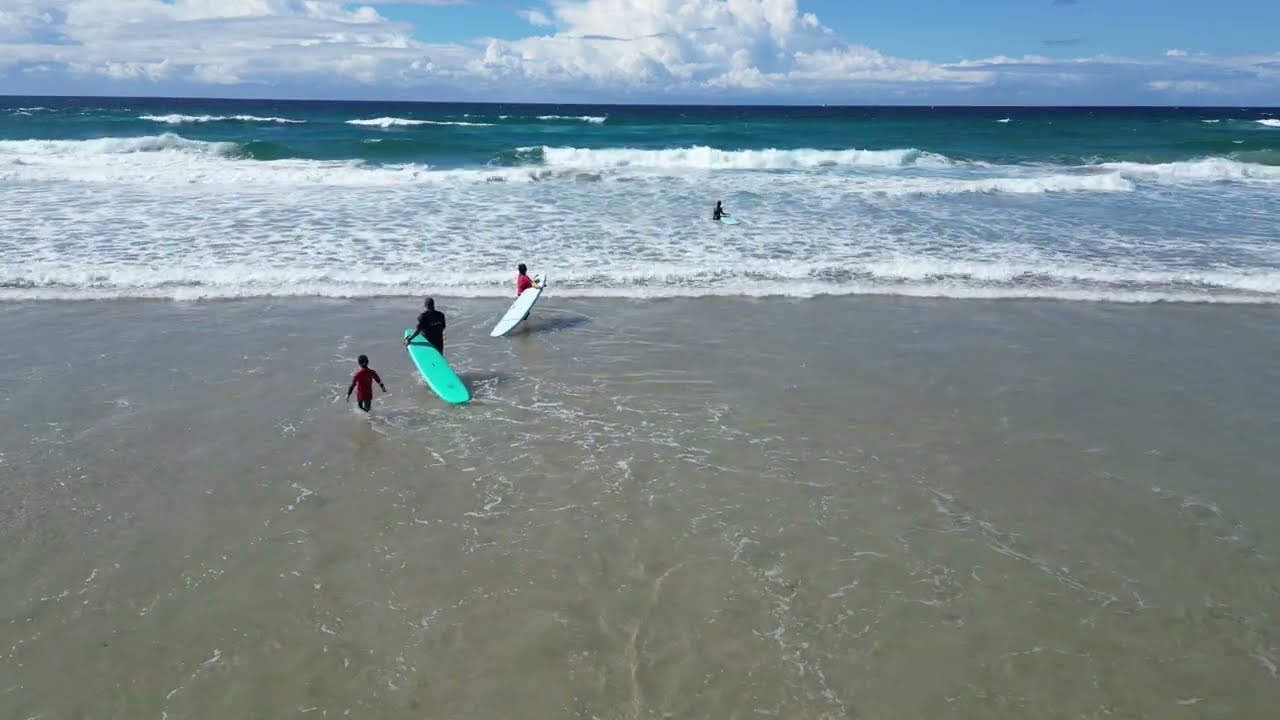The photograph captures a vibrant beach scene on a sunny day with a mix of cloud cover and bright blue sky. The waves are plentiful, crashing onto the dark brown sand, creating white, foamy water in the shallow area. The ocean transitions from a turquoise hue near the shore to a dark bluish-green in the distance. The primary focus of the image is on four individuals. One person, dressed in dark clothing, is positioned waist-deep in the water, standing next to a surfboard. Near the shoreline, two adults walk toward the deeper water, each carrying a surfboard—one white and the other a light aqua blue-green. They are joined by a child, who trails behind, walking without a surfboard. The composition showcases the dynamic interaction between the figures and the powerful, choppy waves, set against a picturesque backdrop of a vast, colorful ocean and a sky dotted with substantial white clouds.